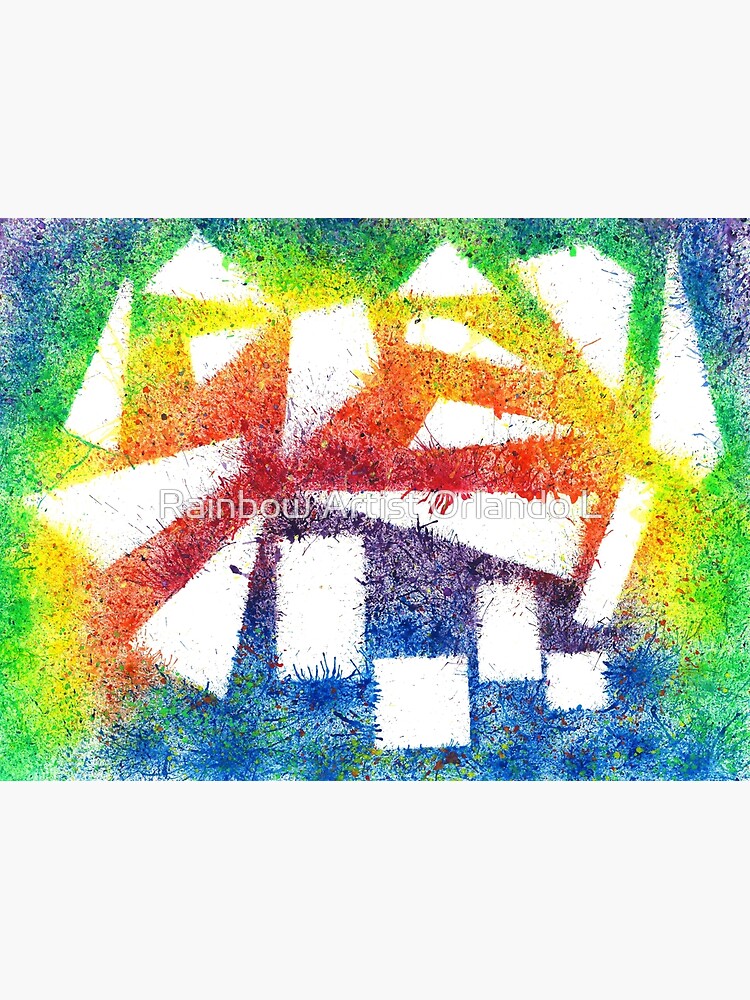This artwork, titled "Rainbow Artist" and created by Orlando L., features a multicolored abstract design with a prominent rainbow theme. The image displays a gradient that transitions from blue and purple at the edges through green, yellow, orange, and red towards the center. The colors blend and splatter in an organic, non-uniform manner. Distinct geometric shapes—squares, rectangles, triangles, and trapezoids—are scattered throughout the composition. These shapes appear to have been masked off during the painting process, creating striking white cutouts that contrast sharply with the vibrant rainbow hues. Some color seepage into the cutouts adds a dynamic, imperfect element to the overall design. The artist’s watermark, "Rainbow Artist Orlando L.," is centrally placed, emphasizing the creator’s identity.